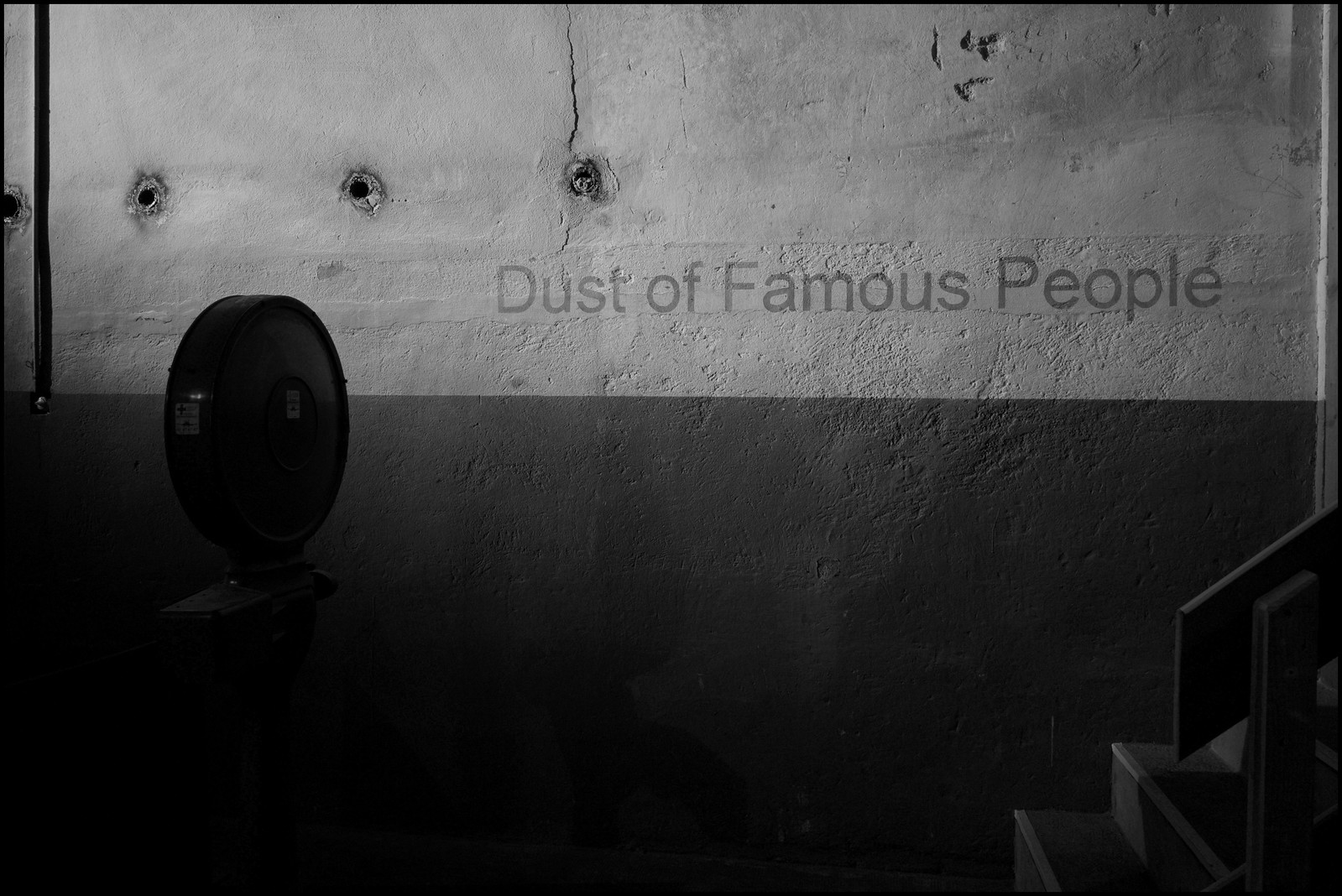The image depicts an old-fashioned, indoor scene in black and white, likely of a mausoleum or a part of a ship, characterized by a light gray wall inscribed with the words "Dust of Famous People" in dark gray or black. The wall shows various imperfections, including three bullet holes along the bottom and additional dents, scratches, and cracks that add to its aged appearance. To the right, a narrow staircase appears to lead into a room, and there is an urn positioned in front of the wall, suggesting a place for collecting ashes. Additionally, a film reel can be seen off to the side of the composition, adding to the intriguing and somewhat mysterious context of the setting.